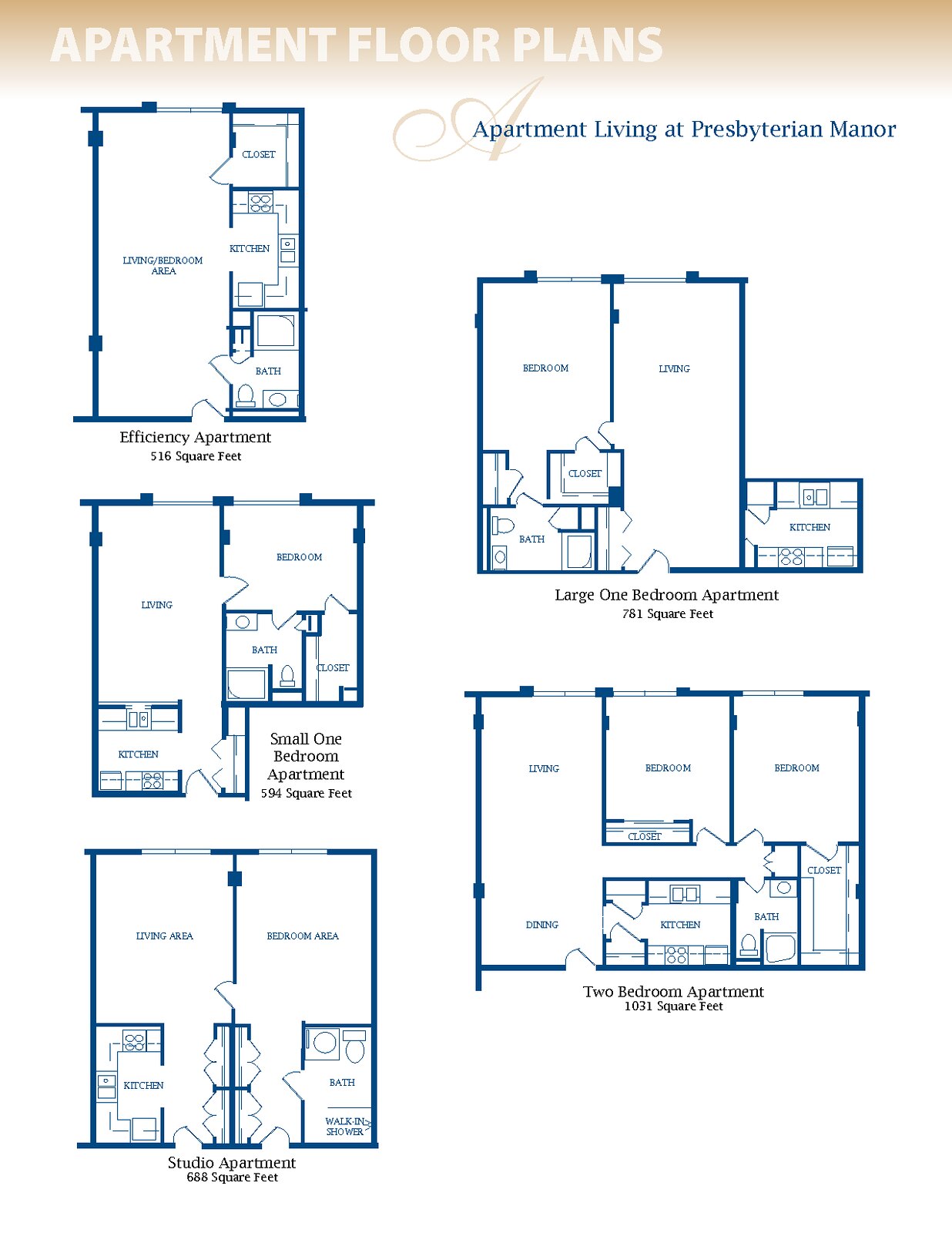This image is a digital photograph, appearing as though it has been lifted from a website, showcasing various apartment floor plans for an apartment complex. The plans, categorized from efficiency to two-bedroom units, are displayed under a banner that features a gradient of whitish, reddish, and orange hues. In bold white font, it reads "Apartment Floor Plans." A decorative heart with a swirling design in lighter gray font is situated more to the right. Below it, in blue text, the complex’s name, "Apartment Living at Pespertarian Manor," is prominently displayed.

Starting from the upper-left corner, the efficiency apartment is depicted as a compact and square layout measuring 516 square feet. It features a closet in the upper right corner, a kitchen, a bathroom, and an open living area. This plan is labeled "Efficiency Apartment" in black text.

Directly beneath it is the small one-bedroom apartment, occupying 594 square feet. The entryway leads to a kitchen immediately on the left, which flows into a living room. The bedroom, positioned on the right side of the living room, includes a sizable walk-in closet and a neighboring bathroom. This layout is marked "Small One Bedroom Apartment" in black text.

Next, the studio apartment, intriguingly designed with two entry doors, spans 688 square feet. Entering from the left door places the kitchen on the left side and two coat closets on the right. The living area is centrally located, with a dividing door leading into the bedroom area. Opposite the closets, a bathroom is situated along the right wall. This is denoted as "Studio Apartment" in black text.

Following is the large one-bedroom apartment, which covers 781 square feet. Upon entry, a spacious living room greets you, with a protruding kitchen on the right. This transition into a bedroom features an expansive walk-in closet, an additional smaller closet, and an adjacent bathroom. This configuration is identified as "Large One Bedroom Apartment" in black text.

Lastly, the two-bedroom apartment, the largest of the floor plans, encompasses 1,031 square feet. Entry into the unit leads directly into the dining area, which is contiguous with the living room. A hallway guides to the first bedroom and up to the sizable master bedroom, which houses a large walk-in closet. Returning from the master bedroom, the bathroom is positioned across the exterior wall. Near the front entrance, one finds the entrance to the galley kitchen. This layout is indicated as "Two Bedroom Apartment" in black text.

Overall, these detailed floor plans offer a comprehensive view of the varied living spaces available at Pespertarian Manor.